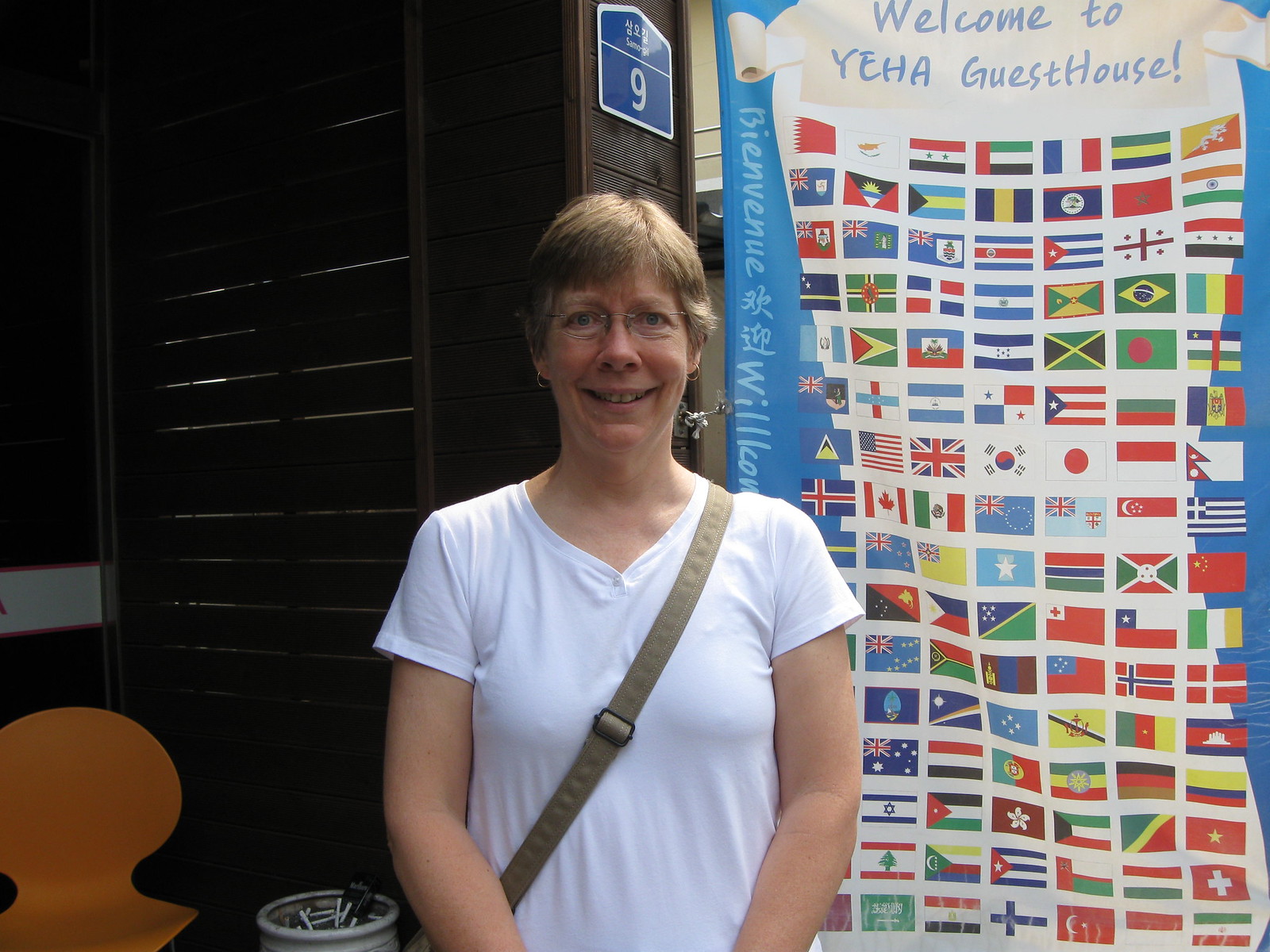In an indoor setting, a smiling woman with short blonde-brown hair, glasses, and a white v-neck t-shirt stands in the center of the image. She has a crossbody bag strapped over her shoulder. The backdrop includes a prominent banner on the right side that reads "Welcome to Yeehaw Guesthouse" in blue font, festooned with dozens of small, colorful country flags. The banner also features greetings in different languages, including "Bienvenue" and "Willkommen". Behind the woman on her left, there's a small gray container filled with items, possibly cigarette butts, inside a bucket. To her left, an orange plastic chair is visible at the bottom corner of the image. Additionally, a small sign with the number nine is mounted on the wall behind her. The atmosphere suggests a European hostel or guesthouse, hinting at a vacation setting.